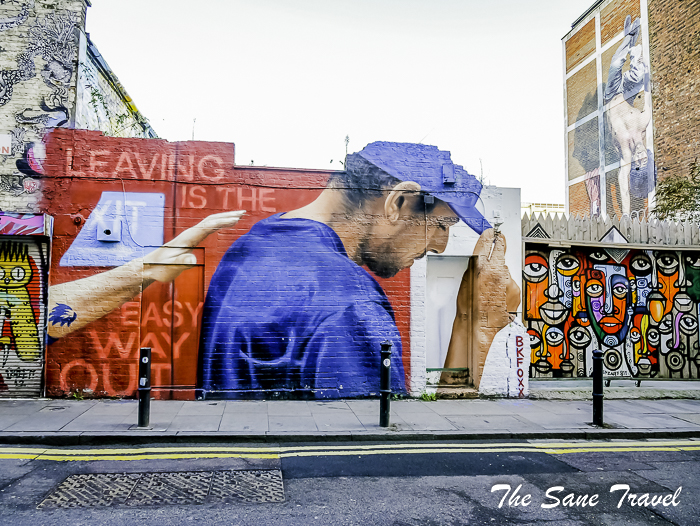The photograph captures an urban street scene vibrant with diverse murals. At the center, a compelling mural in red, blue, and white depicts a man with a beard wearing a blue baseball cap and blue t-shirt, tipping his hat downward. Behind him, a hand stretches out as if reaching to touch him. The mural features bold block lettering that reads, "Leaving is the easy way out," and includes a partial blue exit sign pointing toward the man. 

Adjacent to this central mural are more colorful and cartoonish artworks. To the left, a scrolling metal fence displays a picture of a cartoon bird. To the right, bright and abstract Picasso-like figures fill another mural with disjointed eyes, noses, and mouths. Nearby, a topless figure flipping backward in hues of orange, black, and blue catches attention. 

Above and around these key pieces, additional buildings adorned with graffiti extend the urban art scene. 'BKFOXX' appears in significant lettering beside the central image, lending the artist's signature touch. The street itself, with bollards protecting the murals, adds an authentic urban context to this vivid tapestry of street art.